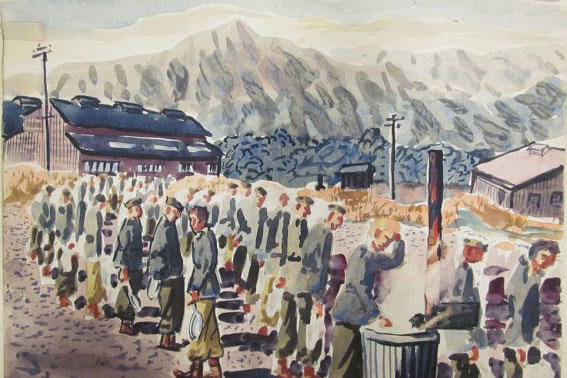This watercolor painting portrays a somber scene of a Nazi concentration camp during World War II. In the foreground, a large group of prisoners, all dressed in identical gray uniforms, are shown lining up, many holding dishes or pans, suggesting they might be waiting for food. To the bottom right, a few prisoners linger near a silver trash can, reminiscent of desperate times. The background is dominated by crude buildings: a large, red-brick structure with a black roof, identified as the shower house, stands on the left, while other utilitarian buildings stretch across the scene. Power lines extend from the buildings, and a smokestack rises ominously. Beyond, the setting is framed by gray mountains under a cloudy sky, enhancing the bleak atmosphere.